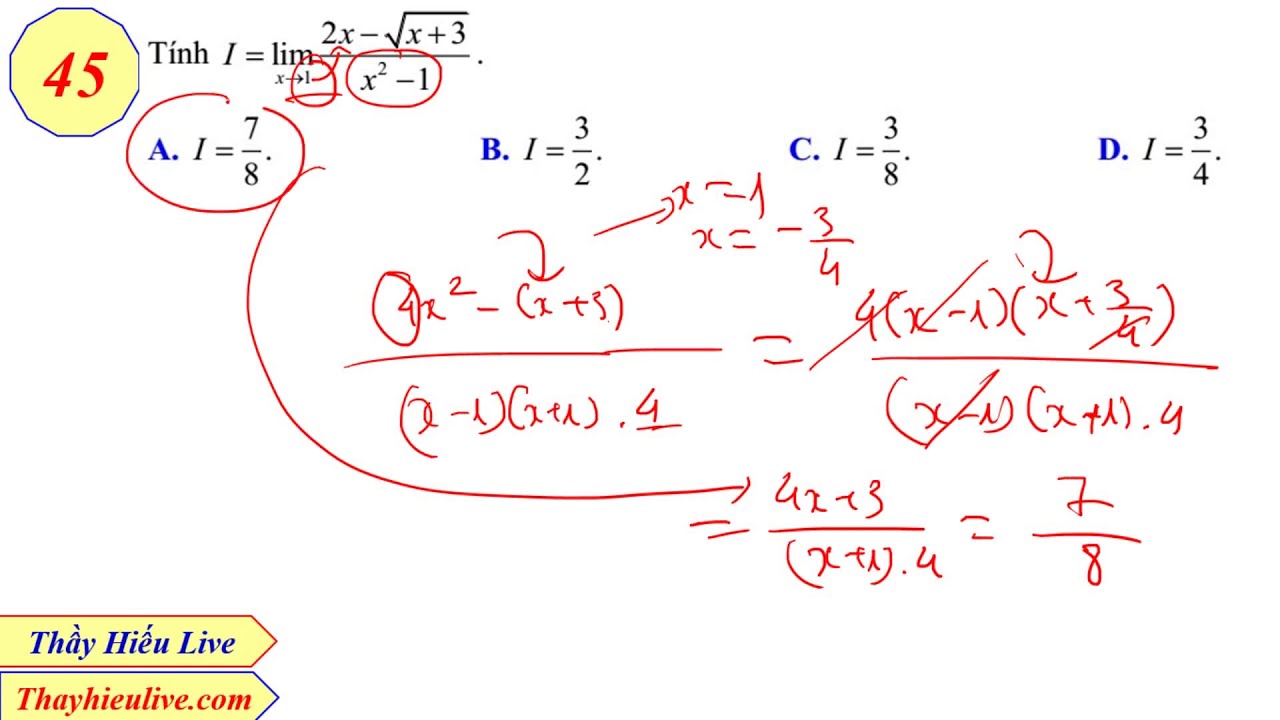The image depicts a mathematical problem being worked out on a digital tablet with a white background. In the upper left, there is a yellow octagon with the number 45 in red font and a blue outline. Below it, there are yellow arrows pointing to the website thayeulive.com, written in red and blue text. The main focus is a mathematical problem written in red pen, surrounded by several annotations and hand-drawn elements. The problem reads "10i = lim (2x - √(x + 3)) / (x → 1) (x² - 1)," and is followed by four options: A) i = 7/8, B) i = 3/2, C) i = 3/8, and D) i = 3/4. The solution has been circled in red, indicating that answer A (i = 7/8) is correct. The image also includes stylized elements like arrows pointing to various parts of the problem and colored circles around key details.